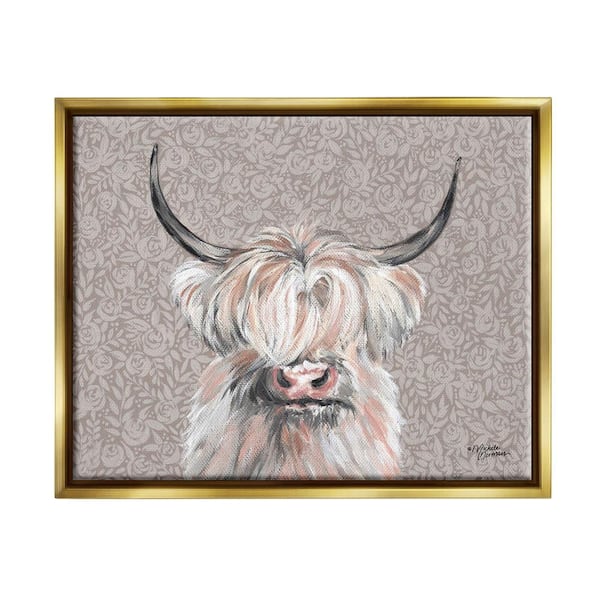The image is a detailed drawing of a large, fur-covered creature, most likely a musk ox, depicted with long, ombre fur in shades of brown, white, and black. It has prominent black horns that curve upward to the left and right. The animal's facial features are partially obscured by its thick fur, with only its pink nose and mouth visible. The eyes are not visible. The background is a beige and brown pattern with rose-like floral textures, adding a soft, natural ambiance. The picture is framed with a gold frame that has an inner brown border. In the lower right corner, there is an artist's signature, though it is not easily readable. The overall aesthetic of the image is enhanced by the blend of realistic and artistic elements, along with the sophisticated frame, which may have been added post-processing for a more elegant finish.